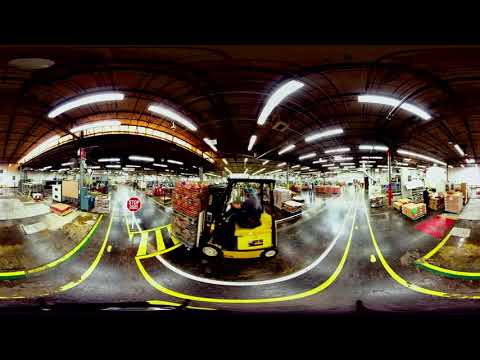The image, taken with a fisheye lens, shows the interior of a large and brightly lit warehouse. At the center of the picture, a person with gray hair, dressed in a black outfit, is operating a small yellow forklift. The forklift is carrying a fully loaded pallet that appears to be filled with materials, possibly with a layer of what looks like oranges on top. The operator is driving down a glossy, paved aisle marked with yellow and white lines for safety. Visible up ahead is a stop sign positioned in the middle of the lane, highlighting the warehouse's safety measures, which include the designated driving path. Surrounding the central aisle, rows of neatly placed pallets create an organized environment. In the background, one can see additional people walking around and more pallets stacked in rows. The tall ceiling, composed of wooden planks and equipped with large tube lights, is curved due to the fisheye effect, adding to the spacious ambiance of the warehouse.